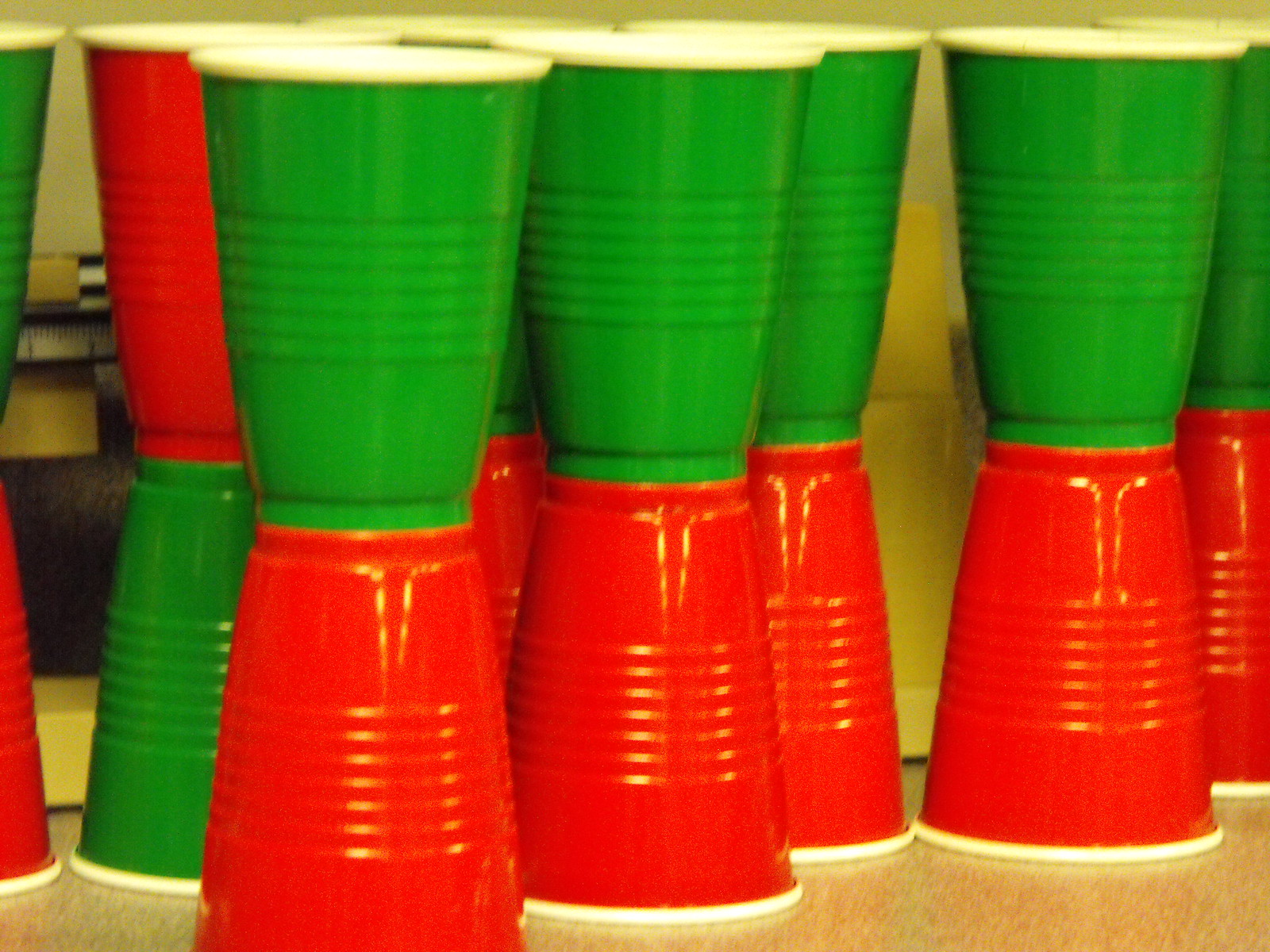The photograph features an intricate arrangement of red and green plastic Solo cups, characterized by their white interiors and rims. The cups are stacked in pairs, with several sets showing a predominantly red cup flipped upside down at the bottom, and a green cup positioned upright on top of each red cup. This creates a striking Christmas color combination. Additionally, there is one pair where the orientation is reversed, with a green cup at the bottom and a red cup on top. The cups are designed with a ribbed detailing about halfway up, enhancing grip. In the background, partially visible, is a yellow kitchen appliance, presumably a stove, with a black window where the oven would be.